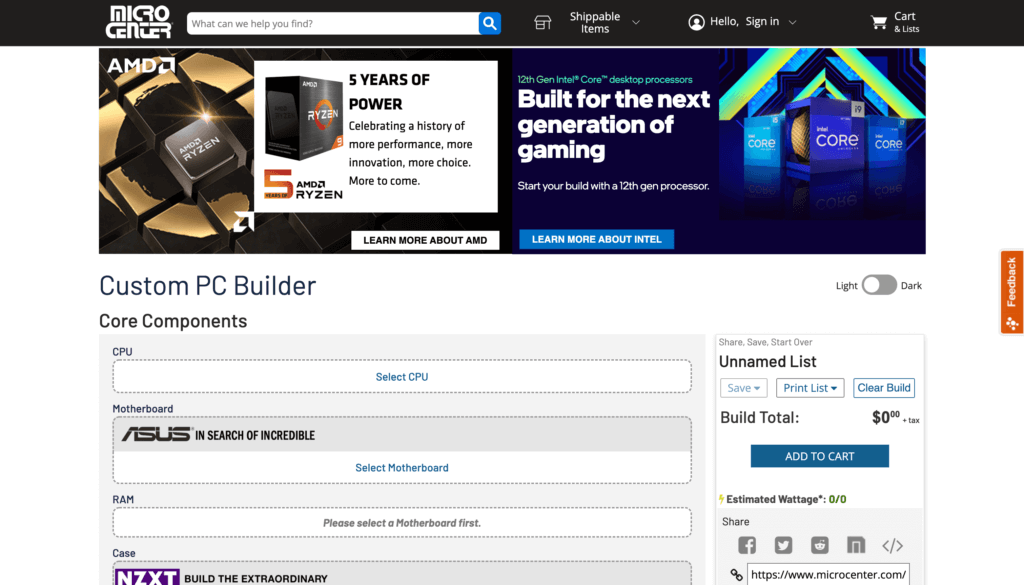Caption: This image is a detailed screenshot of a web page from Micro Center. At the very top, there is a black bar with the Micro Center logo in a futuristic white font on the left. Adjacent to the logo is a search bar with the placeholder text, "What can we help you find?" followed by a blue search button. To the right of the search bar, there are links for "Shippable Items," "Hello, Sign In," "Cart," and "Lists."

Below this top bar is a prominent banner split into two parts. The left-hand side of the banner features an image likely depicting a gaming fan. Overlaid on this image is a white box that says, "Five years of power. Celebrating a history of more performance, more innovation, more choice, more to come. Five AMD Ryzen." There is also a black box with "Ryzen" written in white, surrounded by an orange circle.

The right-hand side of the banner has a blue background with the text, "12th Gen Intel Core Desktop Processors. Built for the next generation of gaming. Start your build with a 12th Gen processor." Below this, there is a blue box with the invitation to "Learn more about Intel."

The section beneath the banner provides options for customizing a PC build. Displayed prominently in white text are "Custom PC Build" and "Core Components." Below, a grey section is divided into selectable components starting with "CPU" and a button labeled "Select CPU." Following this are options for "Motherboard" with an instruction to select a motherboard first before choosing "RAM," and then "Case."

On the right-hand side of the customization section, there is an area for an "Unnamed list" and notes indicating the current build total as $0 plus tax. A blue "Add to Cart" button is located below this information, with an "Estimated Wattage" display showing "0 out of 0."